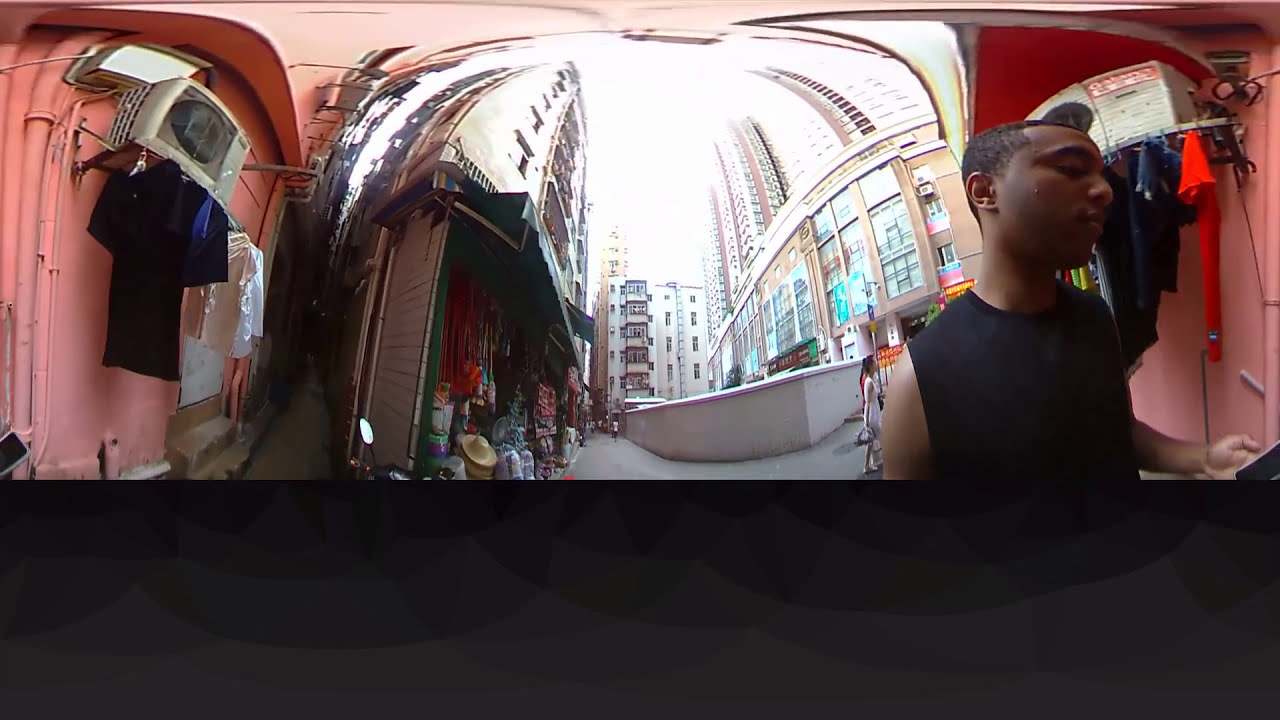In this image taken from what appears to be a ring or doorbell camera outside a building in a foreign city, a man with dark skin and very short curly hair stands to the right, wearing a black tank top and looking at his phone. To his right and in the background, items of clothing in various colors such as red, green, yellow, and black hang on a rack next to a pink wall with an air conditioning unit above. Across from him, in the same doorway, another clothing rack with a black and a white item is visible. The scene extends into a courtyard surrounded by tall buildings, with several stores featuring open doors displaying hats, colorful fabrics, and decorative items. Signs with red backgrounds and yellow writing appear over some of these stores. Nearby, a woman in a white dress stands amidst the bustling market atmosphere, which features the lower floors as bazaars and the upper floors as residential balconies.